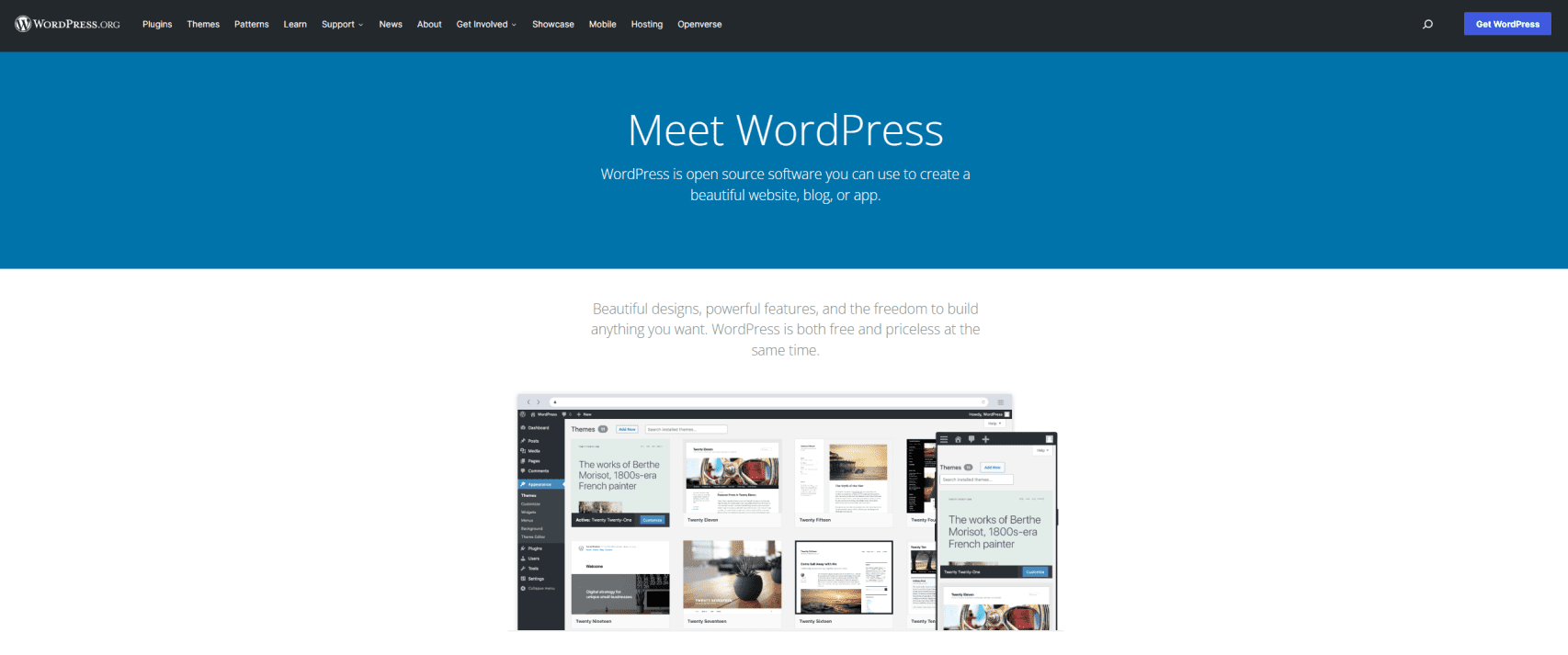This screenshot captures the homepage of the WordPress.com website. At the very top, there is a sleek black navigation bar with white text displaying the menu options: "Plugins," "Themes," "Patterns," "Learn," "Support," "News," "About," "Get Involved," "Showcase," "Mobile," "Hosting," and "Openverse." To the far right, there is a search function, accompanied by a striking blue button labeled "Get WordPress" in white font.

Just beneath the navigation bar, the main section of the page features a bold header reading "Meet WordPress" in white text set against a blue background. Below this, an informative subheading in white font states, "WordPress is open-source software you can use to create a beautiful website, blog, or app."

Further down, the background transitions to white, presenting the text, "Beautiful designs, powerful features, and the freedom to build anything you want. WordPress is both free and priceless at the same time." This inviting message emphasizes the platform's versatility and accessibility.

Centrally located, there is a visual showcase featuring eight distinct patterns, each displayed in individual squares. This array illustrates the diverse layout and design options available to users. Additionally, an image of a mobile phone is prominently displayed, highlighting the platform's mobile optimization capabilities.